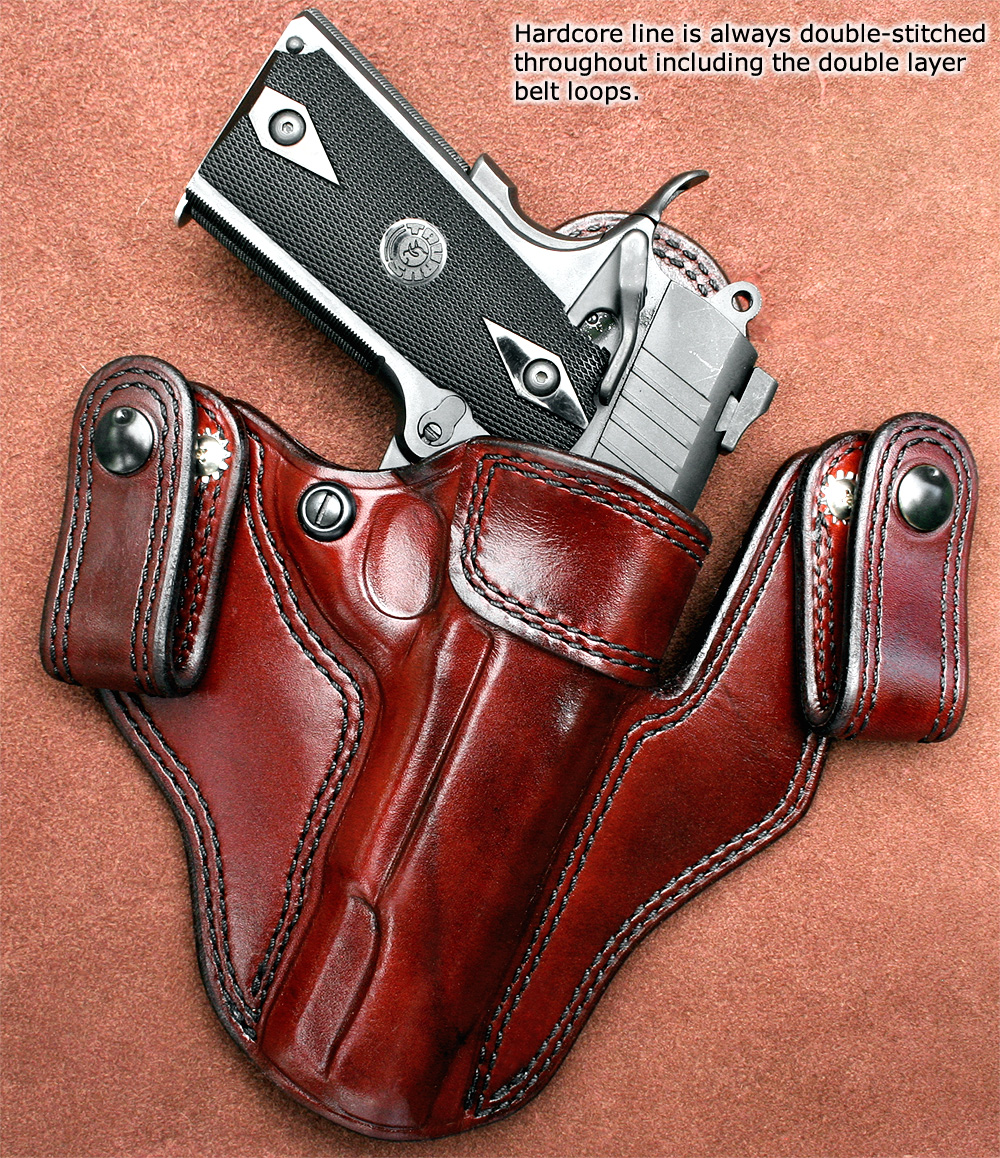The image depicts a compact, semi-automatic pistol with a black textured grip and a brushed silver finish, nestled in a high-quality reddish leather holster. The holster, which features strong, double-stitched seams and double-layer belt loops with black snaps, is prominently highlighted against a rough, textured surface that appears to be a pinkish-salmon, almost orange, outdoor table or stone. The upper right corner of the image bears a caption in black letters that reads, "Hardcore Line is always double-stitched throughout, including double-layer belt loops," indicating that this is a product advertisement for the holster. The overall scene emphasizes the craftsmanship and durability of the holster against the contrasting textured background.